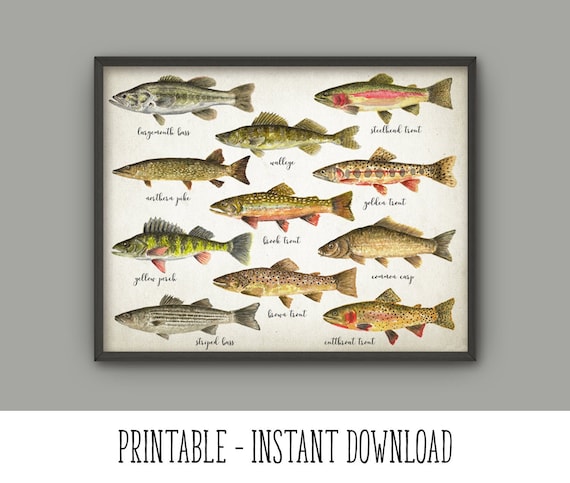This framed artwork, designed as a printable instant download, showcases 11 meticulously detailed illustrations of various sport fish species. Set against a white backdrop, the fish are elegantly depicted with vivid textures and patterns, including stripes and spots, which give a realistic appearance suggestive of colored pencil or acrylic paint techniques. Each fish, ranging from green-hued to gray-toned, is labeled beneath in a cursive script that appears handwritten. Notable species include bass, various types of trout such as brook trout and steelhead trout, yellow perch, and walleyed pike. One of the fish, positioned at the bottom left, is predominantly gray, while another above it displays a striking lime green coloration. Some fish have distinct features like open mouths and notably large red eyes. The entire piece is encased in a black wooden frame and displayed on a gray wall, combining scientific accuracy with artistic elegance.